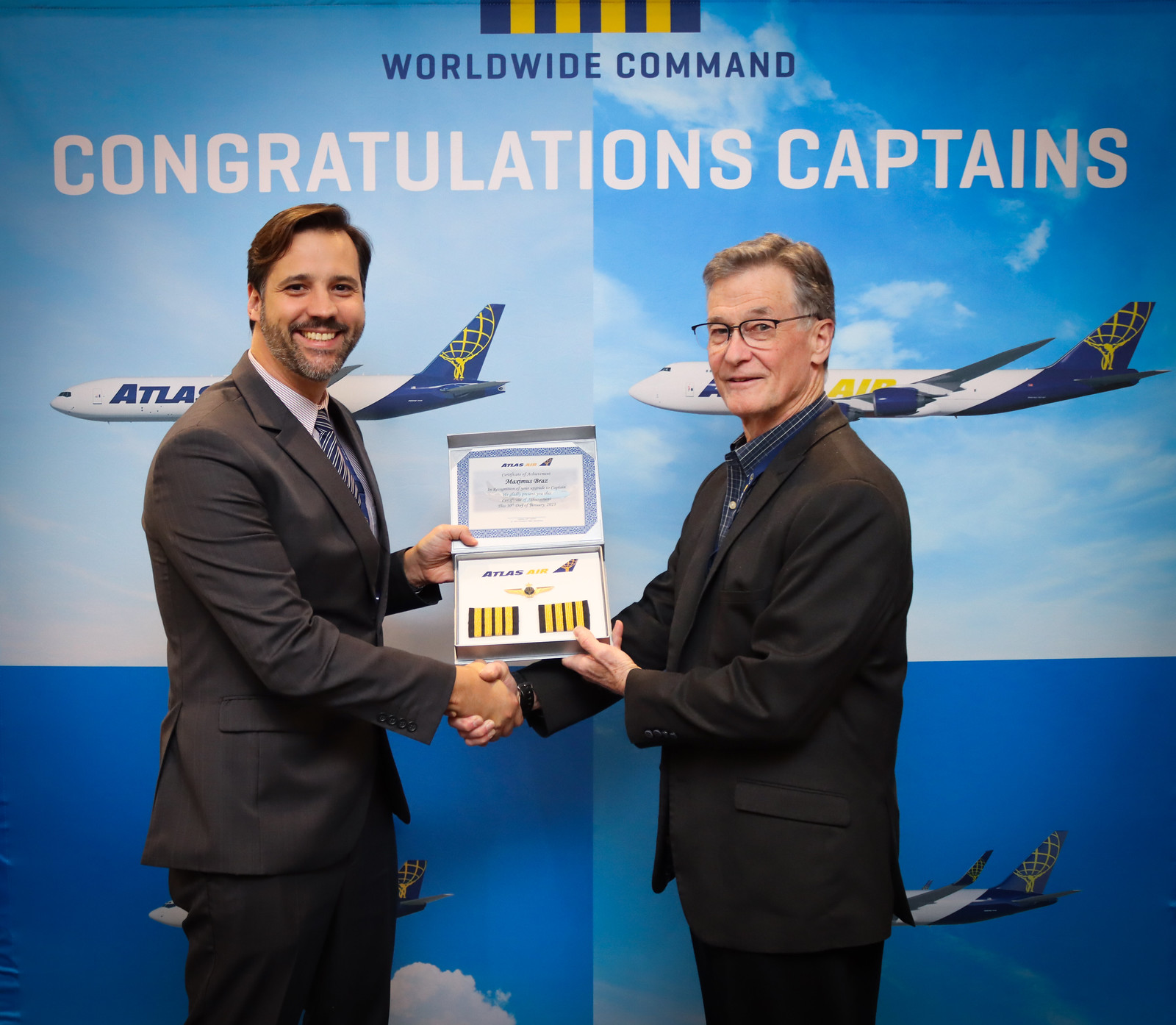The photograph features two white men standing in front of a blue background. The background is intricately designed with a light blue sky, including white clouds and airplanes in both the top and bottom sections. It's segmented into four squares, showing airplanes depicted on both lighter and darker blue skies. The larger text in the background says, "Congratulations Captains" in bold, white letters, with "Worldwide Command" written below in much smaller, black lettering. 

Both men are wearing formal business suits; the slightly younger man on the left sports a tie and has a beard, while the older man on the right, who has glasses, does not wear a tie. They are shaking hands, and each is holding up a certificate together, presumably an award. The man on the right appears to be presenting this certificate to the other.